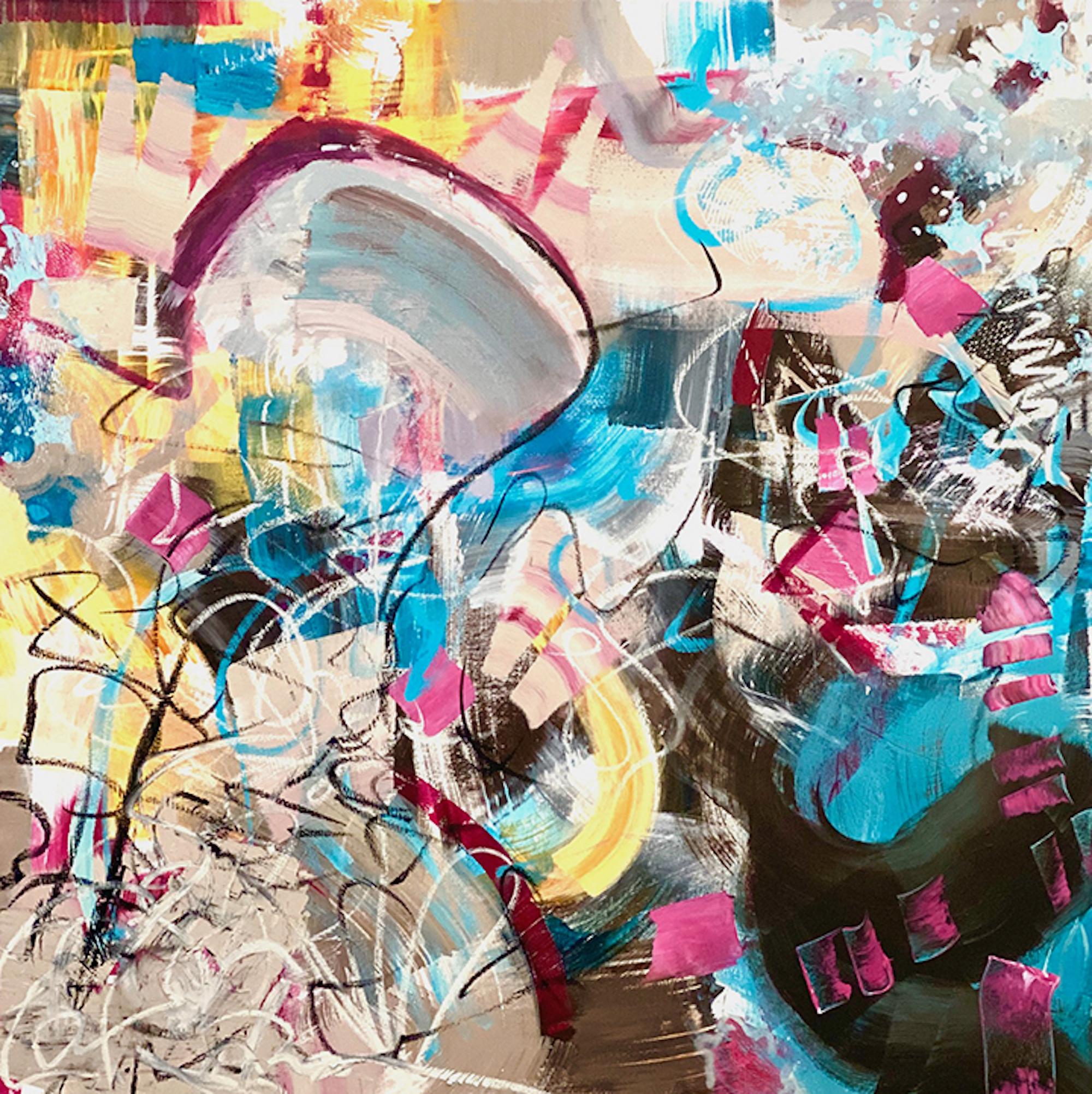This image showcases an abstract painting dominated by vibrant and varied colors. The artwork features an array of yellows, maroons, blues, pinks (both light and dark), whites, and browns, all splashed together without forming any identifiable image. Abundant squiggly marks, notably black and white, crisscross the composition, especially in the bottom half. The black and blue hues predominantly gather in the bottom right-hand corner while gray tones emerge in the top right and bottom left areas. The top left corner is saturated with yellow, with a single yellow swath extending towards the middle-bottom region. An unreadable signature-like scrawl is located at the bottom of the piece. In the upper right, there's an area suggestive of water or waves, adding an additional layer of texture and mystique to this dynamic and colorful abstract painting.